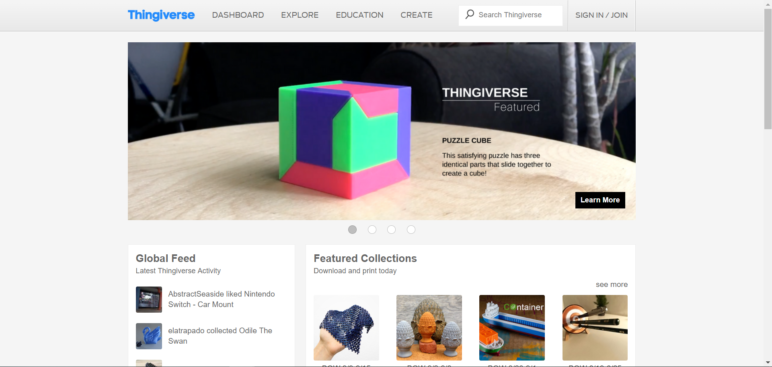In this image, we are viewing a screenshot of the Thingiverse homepage. At the top of the page, the word "Thingiverse" is displayed prominently in blue. Adjacent to this are navigation links in a dark beige color, labeled "Dashboard," "Explore," "Education," and "Create." Below these links is a search bar containing the placeholder text "Search Thingiverse." To the right of the search bar, options for "Sign in / Join" are available.

Under the navigation bar, there is an image of a colorful square box predominantly featuring the colors pink, neon green, and purple. Accompanying this image, the text "Thingiverse" is displayed in white. Beneath this is the underlined word "Featured," signifying this section's importance. The colorful box rests on a light brown wooden table and is labeled "Puzzle Cube." The description below reads, "This satisfying puzzle has three identical parts that slide together to create a cube," printed in black text. On the bottom right of the image box, there is a "Learn More" link.

In the left-hand corner of the page, beneath the main content, the heading "Global Feed" can be seen, followed by "Latest Thingiverse Activity." Below this heading are three thumbnail images. The first is labeled "Abstract, Seaside Light Nintendo Switch Car Mount" though the image itself is unclear. The second shows a blue swan and is titled "Electropodo collected Odie the Swan." The final image box features "Featured Collections," with a tagline encouraging users to "Download and print today." This section includes four small images: a hand covered by a dark blue puppet, a beige face with an orange beak and black beady eyes, two blue chopsticks holding an unidentified object, and a dartboard with three darts piercing its center ring.

The combination of vibrant visuals and detailed navigation options encapsulates the dynamic and creative environment of the Thingiverse platform.